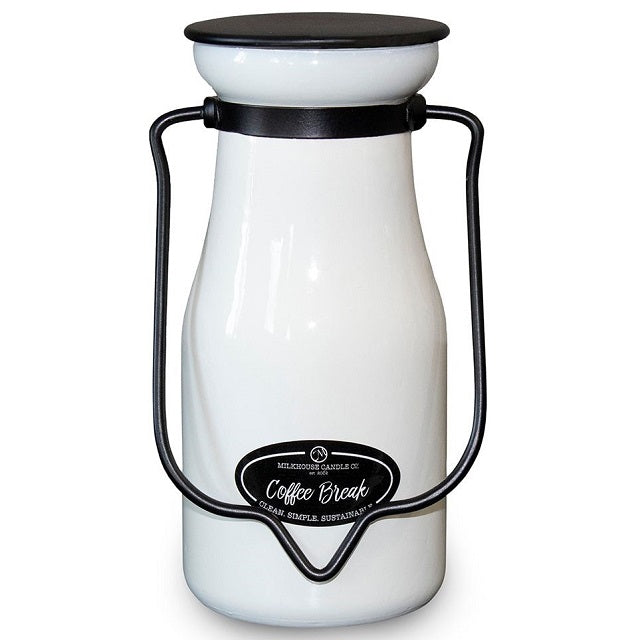The image features a high-quality, white container with black detailing, resembling a porcelain milk carton. The container has a black metal lid and a sturdy black handle, suggesting it might be hung with a candle inside. The lower portion of the container displays a label with the text: "Milkhouse Candle Co., Coffee Break, Clean, Simple, Sustainable." The "Coffee Break" text is in cursive, while the rest of the text is in plain lettering. Additionally, the label features the brand's logo—a circle with a cursive "M" leaning to the right. The overall design is sleek and minimalist, reflecting a blend of practicality and aesthetic appeal.